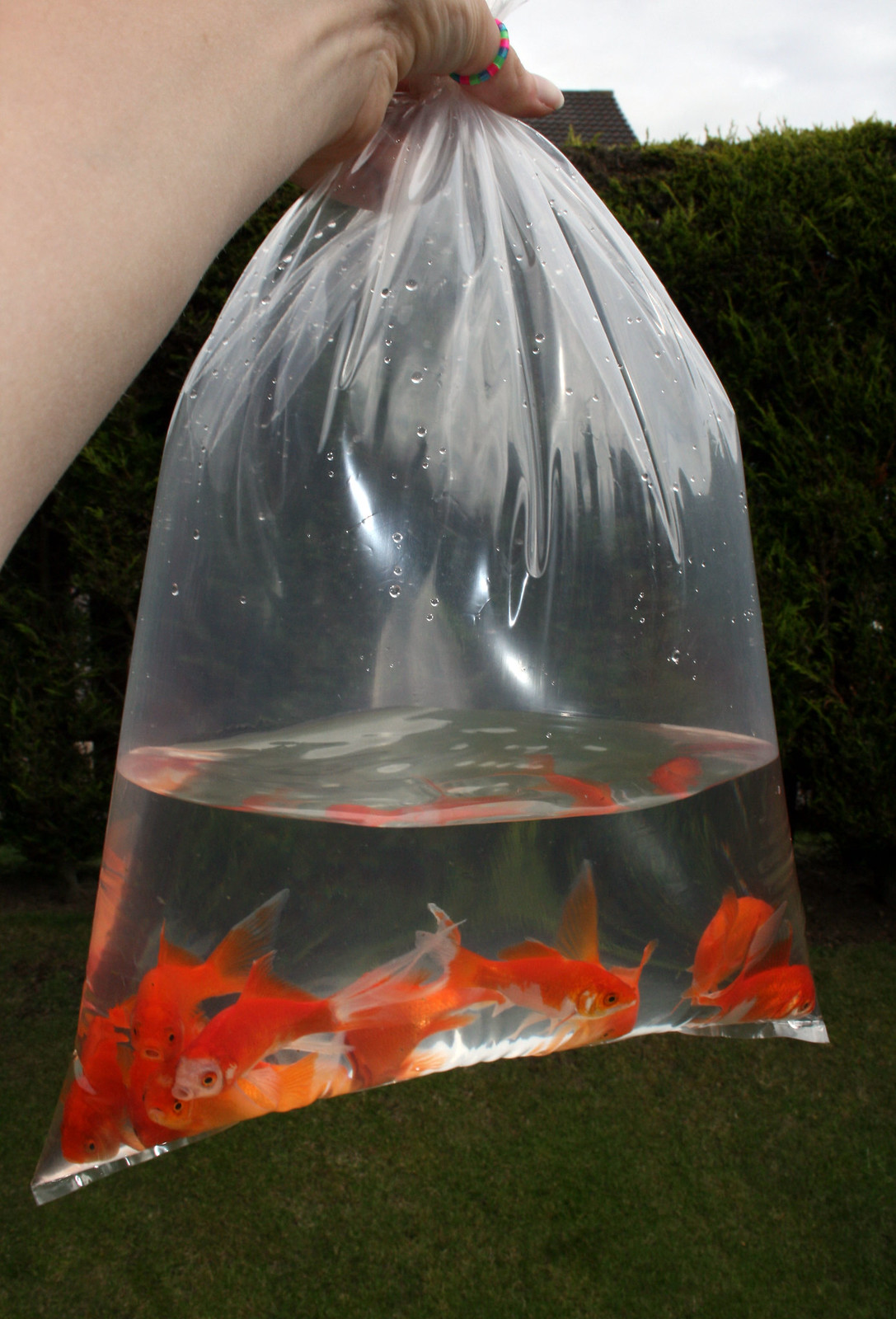This photograph captures a hand prominently displayed, adorned with a distinctive thumb ring featuring green and red, gem-like colors. The hand is holding a clear plastic bag, which is about a quarter to a third filled with water. Within the bag, there are approximately eight to twelve bright orange goldfish, some purely orange, while others exhibit shades of white on their faces or undersides. The goldfish are primarily clustered towards one side of the bag, as if observing the person holding them. The backdrop consists of a meticulously manicured green shrubbery wall and a stretch of dark green grass below, suggesting that the photo was taken in a well-maintained outdoor setting, possibly a backyard. The upper right corner of the image reveals a glimpse of the sky, adding an element of open space to the scene.